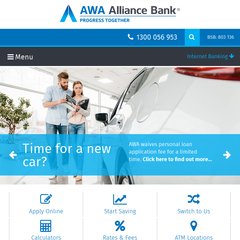The homepage of AWA Alliance Bank features a clear and organized design, dominated by their distinctive branding. At the top, the website prominently displays the bank's name, with "AWA" written in blue and "Alliance Bank" in black. Directly below, the phrase "Progress Together" is elegantly rendered in blue letters beside a sleek blue icon resembling a triangle without its base.

The header also includes convenient features such as the bank's contact phone number and a search bar for easy navigation. Beneath the header, there's a "Menu" button marked by three horizontal lines, which users can click to explore various options.

The main visual attraction in the center of the website is an image of a white car, parked near a tree, with a man and a woman closely examining what appears to be a composition book—possibly reviewing financial documents or learning more about the car.

Overlaying this image, in bold white letters against a striking blue background, is an enticing message: "Time for a new car? AWA waives personal loan application fees for a limited time. Click here to find out more." The call-to-action, "Click here to find out more," accompanied by a directional arrow, invites users to learn more about this special offer.

Towards the bottom of the page, various navigational options are presented, each in blue text with matching blue icons. These options include "Apply Online," "Calculator," "Start Saving," "Rates and Fees," "ATM Location," and "Switch to Us," making it easy for visitors to access the bank's services directly from the homepage.